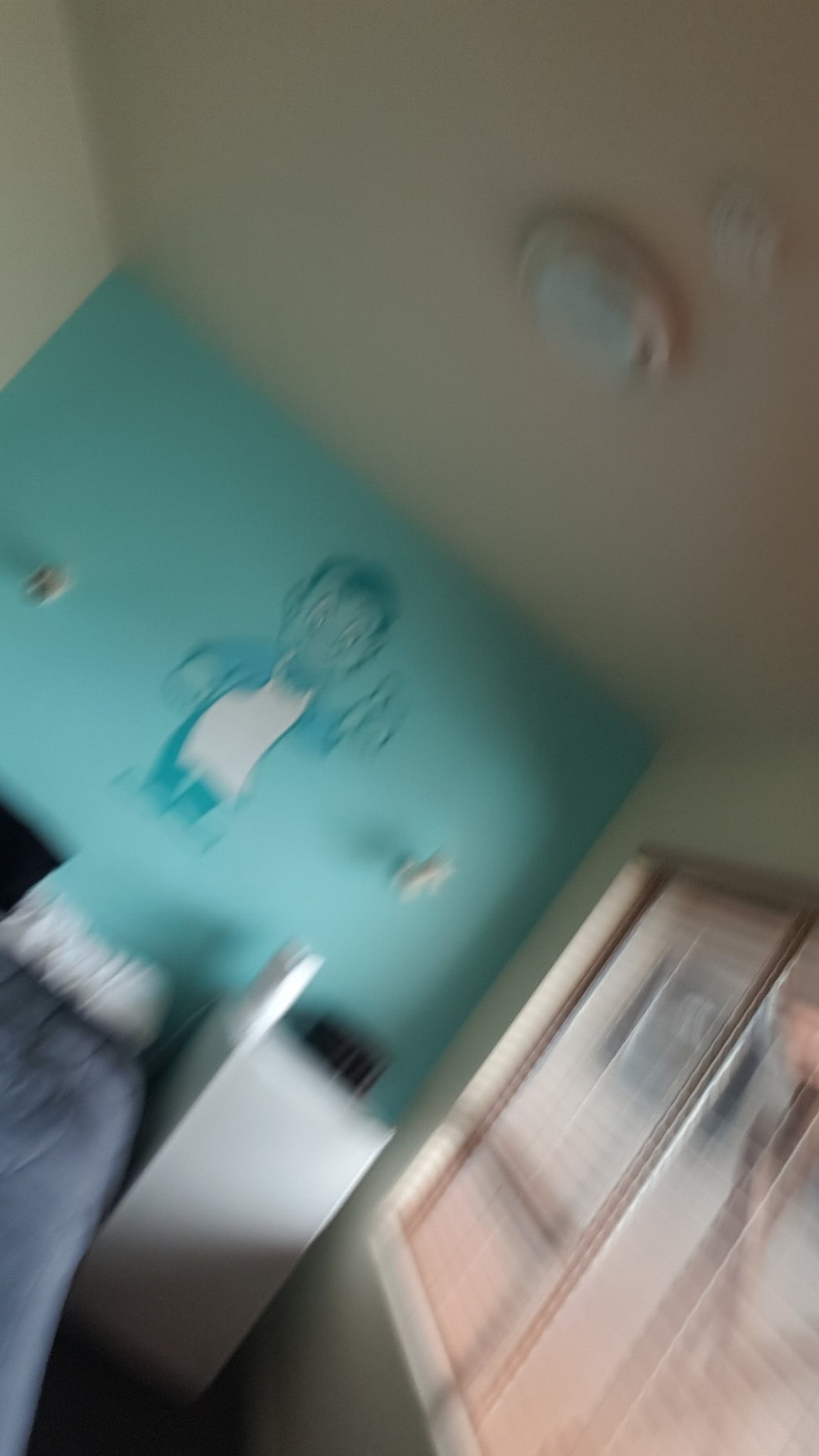The image depicts a slightly disoriented view of a bedroom, captured at a diagonal angle which makes it challenging to perceive straight without tilting your head. The photograph showcases three of the room's four walls. Two of these walls, along with the ceiling, are painted white, and the ceiling features a circular light fixture centrally positioned. The back wall of the room is a light sky blue and prominently displays a large image of the Bob's Big Boy mascot, which occupies approximately half of the wall's surface.

In the left corner of the image, the edge of a bed is visible, adorned with a blue comforter and topped with white pillows. The bed is positioned against the back wall with the light sky blue paint. Adjacent to the bed is a white dresser, contributing to the room's furnishings. On the right-hand side of the image, the right wall features a large window equipped with blinds, allowing for natural light to enter the room.